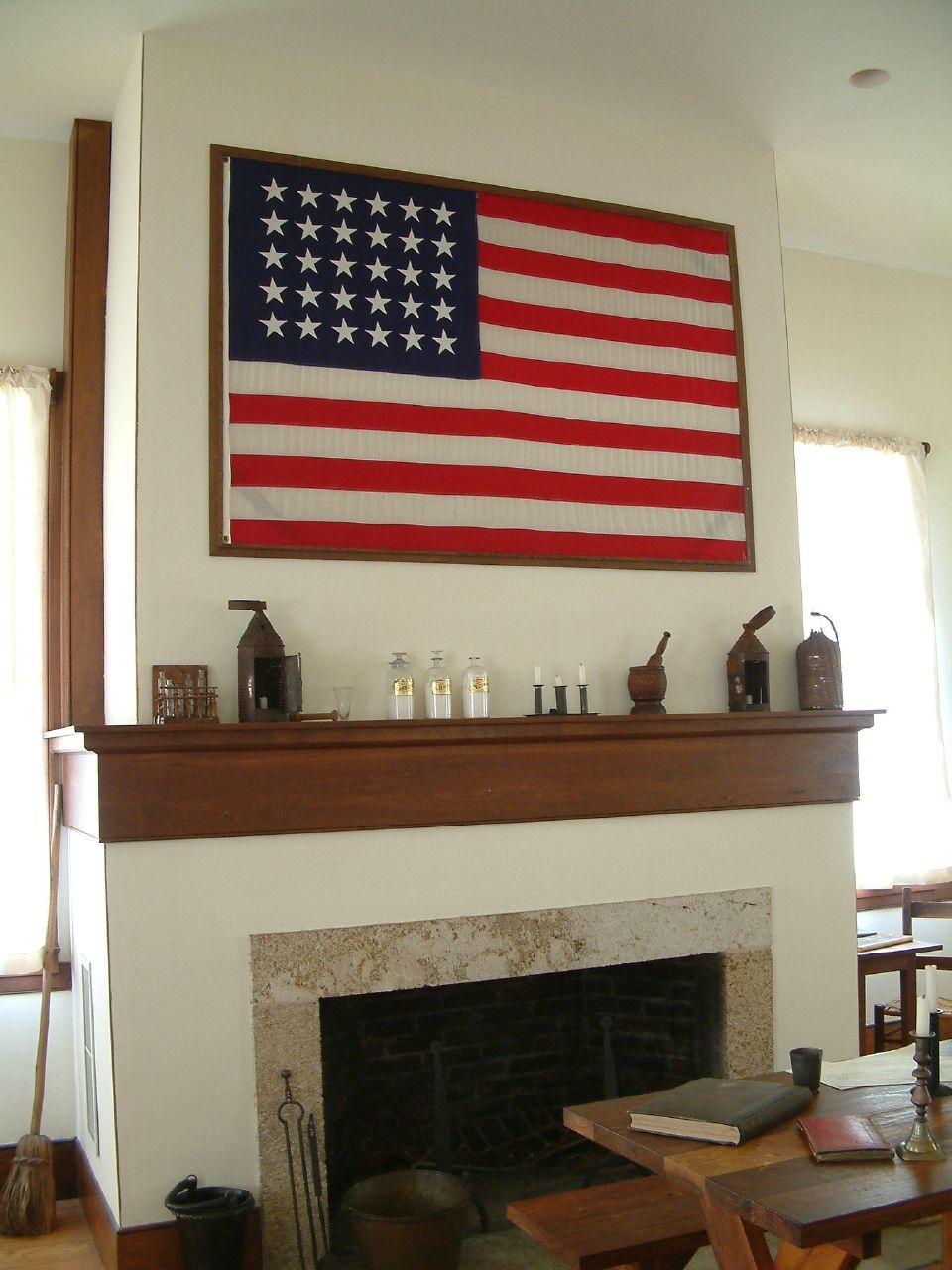The photograph captures an interior scene, possibly from a museum or a historical setting, featuring a prominent fireplace with a wooden mantle adorned with vintage items. Above the fireplace, there is a framed American flag with 30 stars, indicating a period likely between the Civil War and World War I. The mantle displays a variety of antique objects, including candlesticks, a wooden mortar and pestle, and small old-fashioned bottles containing white powder. Leaning against the left side of the fireplace is an old-fashioned broom. The fireplace itself is surrounded by a white material, possibly stone or plaster, while the walls are a cream color. In front of the fireplace is a wooden picnic-style table holding two books, a cup, and two tapered candlesticks. The room features hardwood flooring and white curtains flanking the windows on either side of the fireplace. The overall vividness and details suggest this could be a historical photograph or a meticulously designed period room.